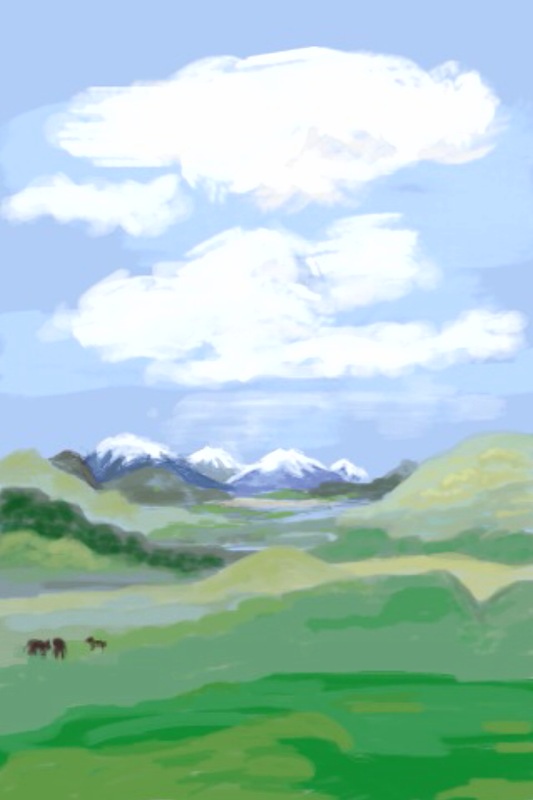This watercolor painting captures a serene mountain landscape with intricate details. Dominating the backdrop are majestic, snowy mountain peaks painted in dark blues and whites. The painting transitions to lush rolling hills in lighter greens, moving forward to a richly green foreground. On the left side of the scene, a group of horses grazes peacefully on the abundant grass. The sky above is a wash of light blue, adorned with soft, white clouds. A subtle yet noticeable river winds its way through the valley, nestled between the hills, enhancing the depth and tranquility of the scenery. The artist's blend of colors and shading techniques masterfully conveys the natural beauty and serenity of this mountainous pasture under a bright, cloud-kissed sky.